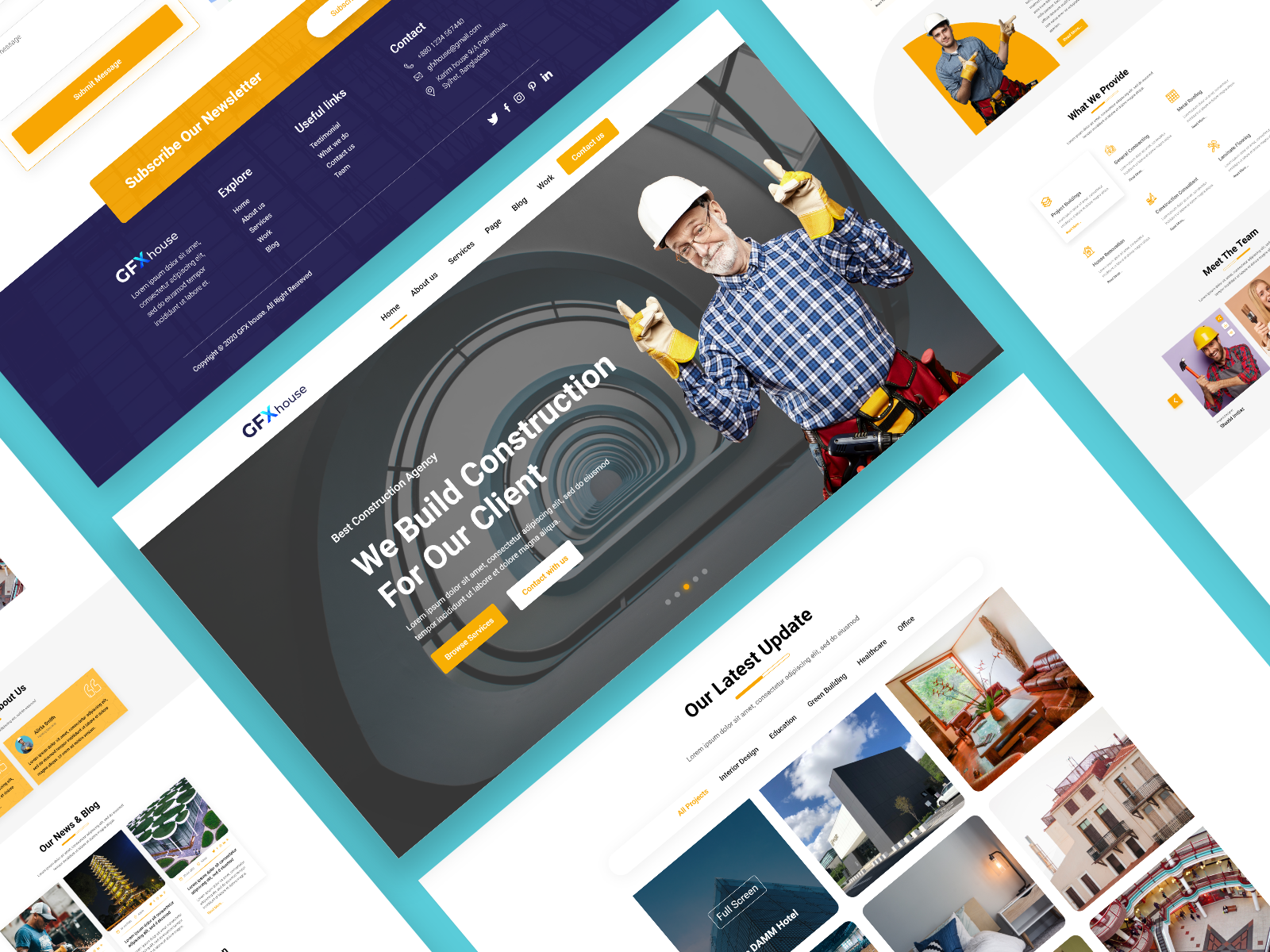Caption: 
A comprehensive brochure for the CFX House features prominently in the image. An orange box invites readers to "subscribe to our newsletter," while a contrasting navy blue box introduces the GFX House with options like "Learn," "Explore," "Home," "About Us," "Services," "Work," "Blog," "Useful Links," "Testimonial," "What We Do," and "Contact Us." The contact section provides a phone number and Gmail address. 

The brochure also highlights the Cream House, including its address and a copyright notice from 2020. A picture of a construction worker wearing a tool belt, yellow gloves, a hard hat, a plaid shirt, glasses, and a beard appears with the caption "Best Construction Agency: We Build Construction for Our Clients." 

Aside from this, there are mentions of various projects categorized under "Interior Design," "Education," "Green Building," "Healthcare," and "Office." Accompanying images illustrate an office, an office building, and a hotel room. The entire layout of the brochure is presented diagonally across the page.